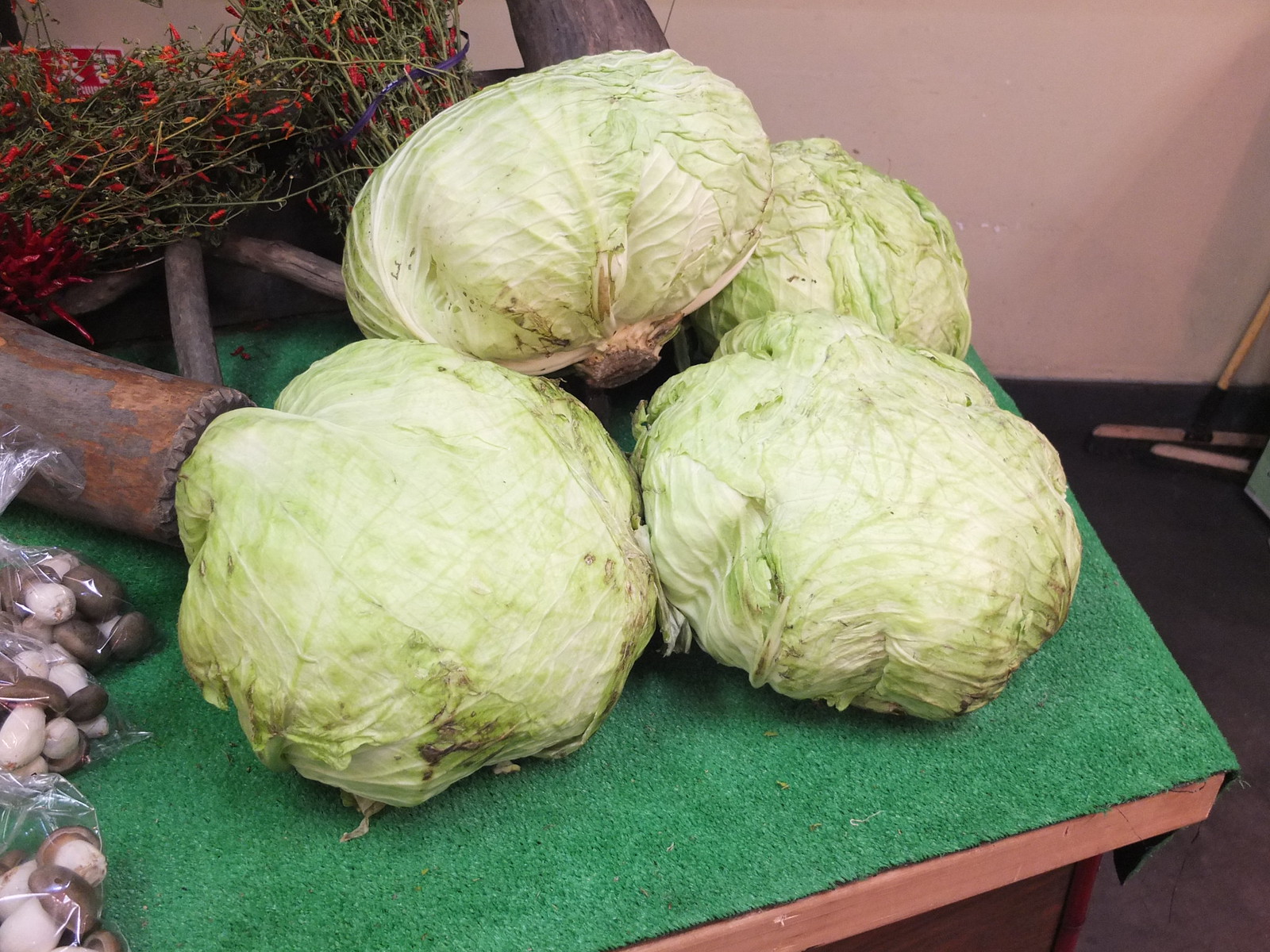This is a detailed photograph featuring a small display of fresh produce on a wooden table covered with a green, velvety-textured cloth that resembles fake grass. The centerpiece consists of four cabbages, three of which are large and one smaller. These pale, nearly white cabbages with light green tinges exhibit a crinkly texture, with tightly wrapped leaves, especially the one on the far left, which is notably round in shape. Adjacent to the cabbages, there are a few bunches of dried-out chili peppers, identifiable by their long, red fruit. To the left side of the cabbages, several bags of what appear to be mushrooms, brown and white in color, are also visible. The setup, likely at a farmer's market, suggests that these organic items are on display for sale, laid out in a somewhat rustic and natural fashion.